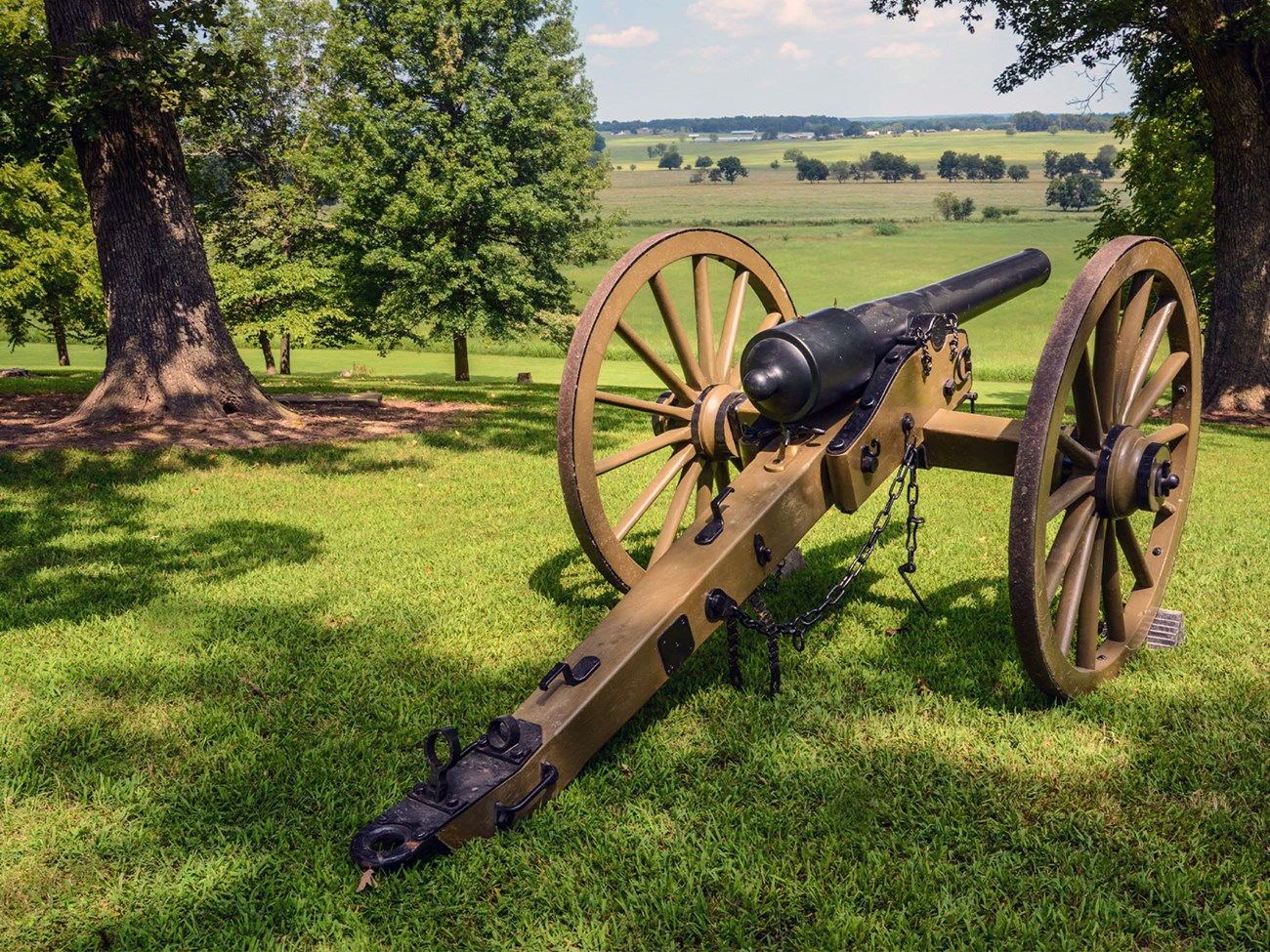This photograph captures a historic, older-style black cannon mounted on a tripod base with large wagon wheels, resting on a grassy hillside. The wheels and base are brown, with visible black hardware including hooks, handles, and chains. The cannon is positioned diagonally and faces away from the viewer. The scene is an outdoor setting, with rich green grass in the foreground, casting tree shadows. To the left, a tree trunk is visible, and more trees with green leaves are scattered in the background, leading to open fields dotted with additional trees. The sky above is overcast, painted in dull gray tones, adding an atmospheric touch to this picturesque and historic landscape.